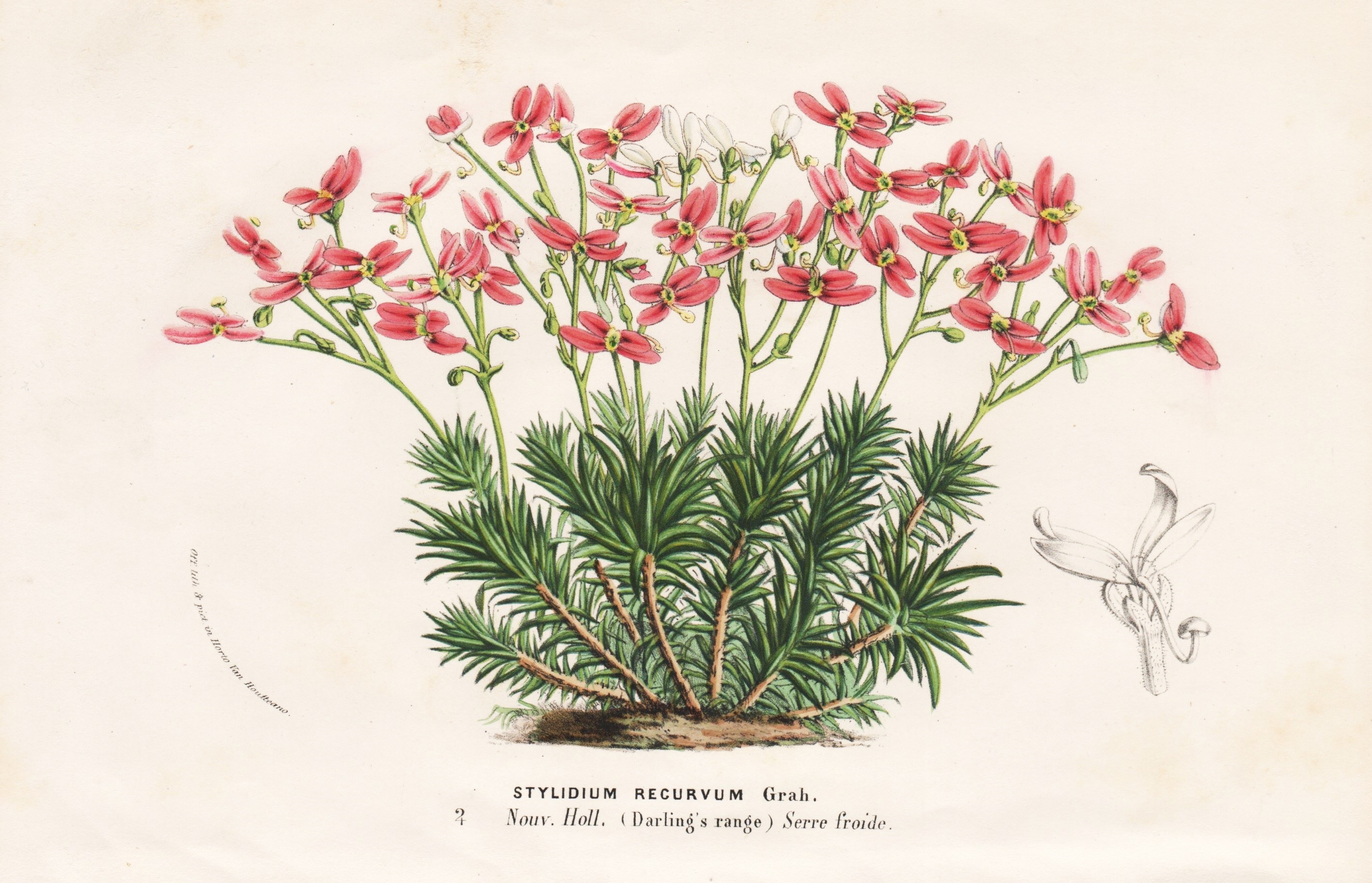The image is an older, color-illustrated botanical drawing of a plant, reminiscent of illustrations from late 19th to early 20th-century nature or botany books. The background is off-white, appearing yellowed with age. The plant, identified at the bottom in bold capital letters, is labeled "Stylidium recurvum Grah." and "Darling's Range" with additional text "nou.v. holl."

The drawing depicts the plant's structure in great detail. At the base, woody stalks emerge from the ground, giving rise to spiky green leaves arranged in clusters, resembling pine needles. These stalks transition into longer, more barren green stems higher up. Each stem is crowned with a reddish-pink flower featuring four petals and a yellow center, indicating the reproductive parts. Adjacent to the main illustration, on the right, is a gray, line-drawn enhanced depiction of the flower's pistil and stamen, providing additional detail.

The overall appearance includes colors such as green, pink, brown, and gray set against the off-white backdrop, complemented with stylized script text on the left side, which remains partially unreadable.